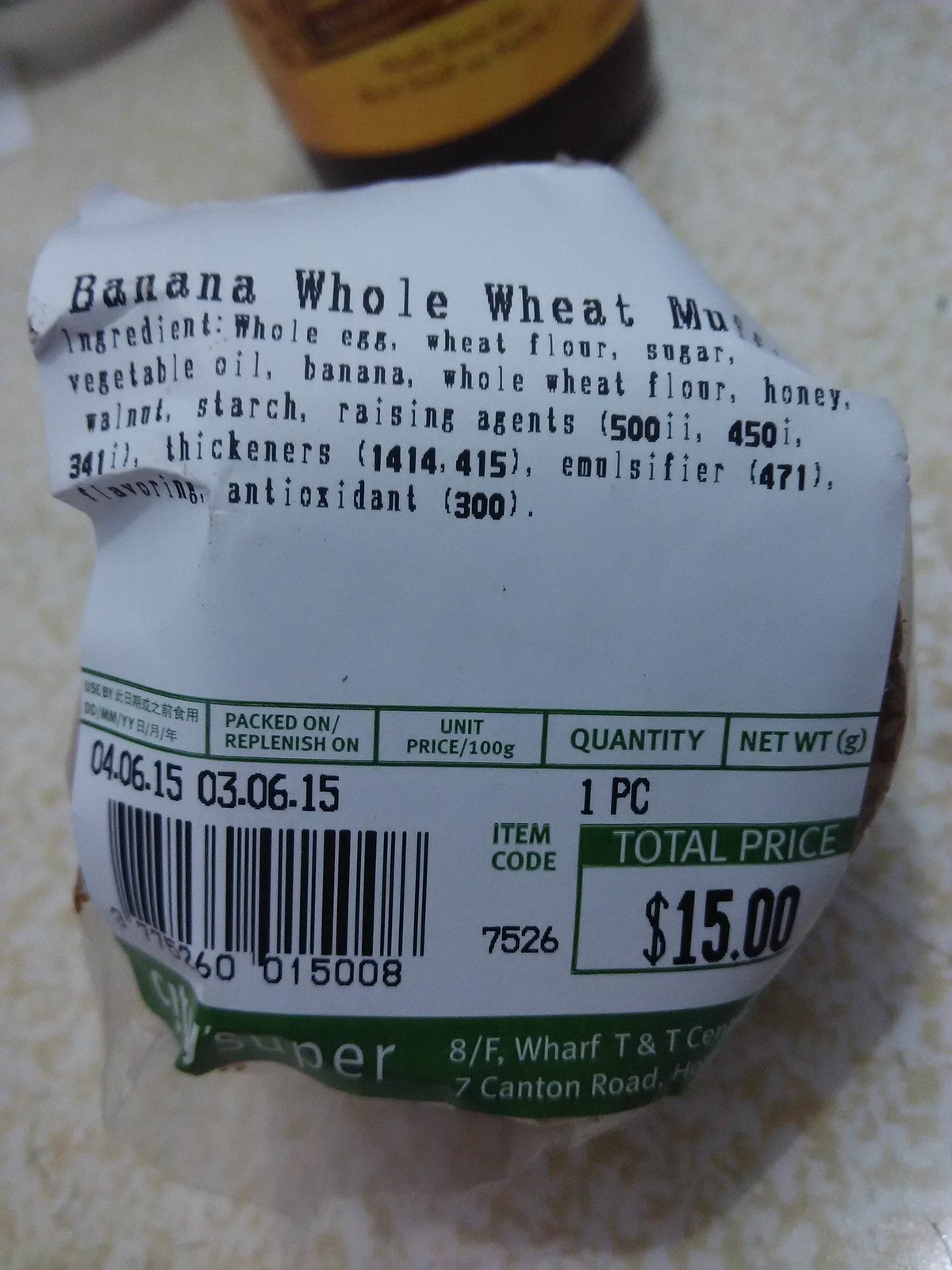This close-up photograph captures a white supermarket label wrapped around a banana whole wheat muffin, partially obscuring its round shape. The label, bent due to the smaller size of the muffin, prominently features the text "Banana Whole Wheat Muffin" at the top, followed by a detailed list of ingredients: Whole Egg, Wheat Flour, Sugar, Vegetable Oil, Banana, Whole Wheat Flour, Honey, Walnut, Starch, Rising Agents (500ii, 450i, 341il), Thickeners (1414, 415), Emulsifier (471), Flavoring, and Antioxidant (300). Printed in black text, the label also includes product-specific details such as the packing date (04.06.15), use-by date (03.06.15), quantity (one piece), and price ($15). Additionally, the label contains a barcode and a green stripe at the bottom with a white-on-green supermarket name "Super" and its address information. The image is set on a white and peach-colored speckled granite countertop, accented with light brown and gold specks. In the background, there is a dark brown jar with an orange label, further enriching the visual composition.